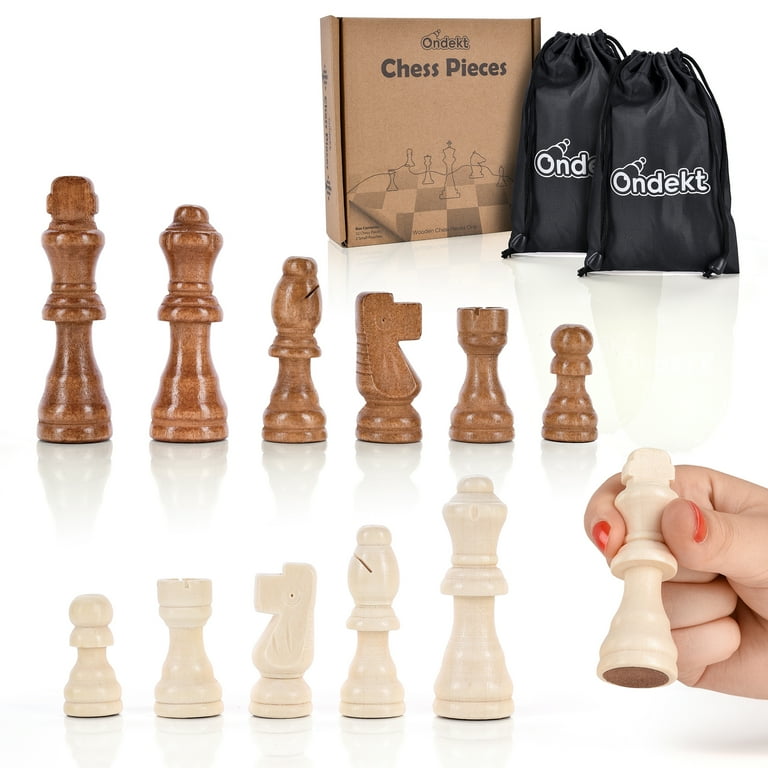The image is a professionally-lit photograph advertising ONDEKT chess pieces. At the top of the image, a brown cardboard box featuring the black text "ONDEKT Chess Pieces" is displayed, along with a detailed black-and-white illustration of a chessboard with pieces. Adjacent to the box are two black drawstring bags with "ONDEKT" imprinted in white letters. Below this section, two neatly arranged rows of chess pieces are displayed. The top row features six medium brown pieces from left to right: King, Queen, Bishop, Knight, Rook, and Pawn. The bottom row mirrors these pieces in a lighter, bone-white color but in reverse order: from left, Pawn, Rook, Knight, Bishop, King, and Queen. In the center of the image, a white hand with peachy coral nail polish prominently holds the white Queen piece, displaying the brown underside of the chess piece. The background is an off-white color, enhancing the clarity and focus of the chess pieces and packaging.